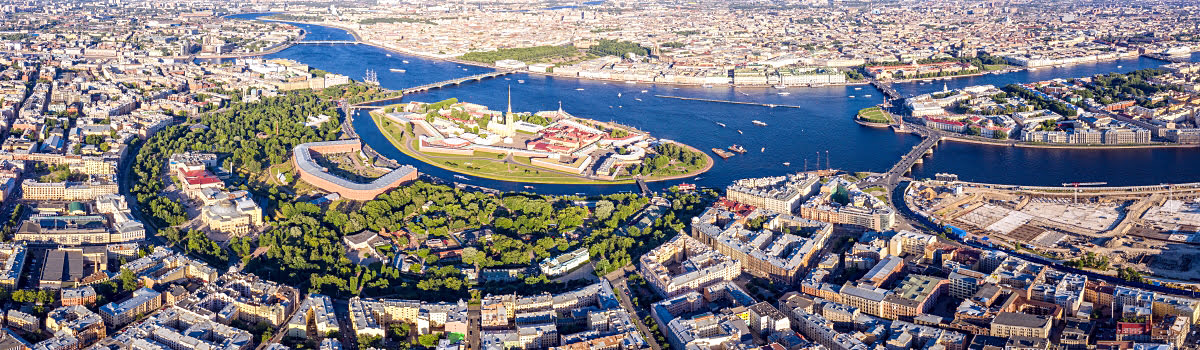This panoramic aerial photograph captures a vibrant, populous city with a large river running through its center. The city is characterized by its dense array of buildings sprawling across both sides of the river. Centrally located within the image is a substantial, lush island, likely a park, surrounded by a canal ring. This island boasts an abundance of trees and features what appears to be a walled structure, possibly a citadel, museum, or government buildings. Multiple bridges span the river, connecting various parts of the city, with one prominent bridge on the right side and another further in the background. The setting is bright and vivid, indicative of daytime. Numerous boats can be seen navigating the river, adding to the lively atmosphere. The architectural details and design suggest that this could be a European city, with characteristic cubed rim areas and courtyard-centered buildings. The image, likely taken with a wide-angle lens from an aerial vantage point, provides a comprehensive and detailed view of this bustling urban landscape.